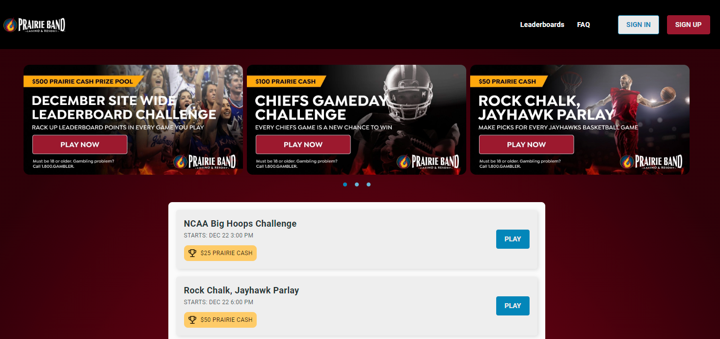**Website Screenshot: Prairie Band Promotions**

In the upper left corner of the website screenshot, the title "Prairie Band" is prominently displayed. Below the title, the navigation menu includes options such as "Leaderboards," "Frequently Asked Questions," alongside a white "Sign In" button and a red "Sign Up" button.

Beneath the navigation bar, the website showcases a series of promotional rectangles:

1. **$500 Prairie Cash Prize Pool Challenge**:
   - **Banner Color**: Yellow
   - **Text**: "December Site-wide Leaderboard Challenge" in white letters.
   - **Description**: Invites users to rack up leaderboard points by playing various games.
   - **Call to Action**: Red "Play Now" button.
   - **Logo**: Prairie Band logo located in the lower right corner of the rectangle.
   - **Image**: Features a picture of a crowd.

2. **$100 Prairie Cash - Chiefs Game Day Challenge**:
   - **Banner Color**: Yellow
   - **Text**: "Chiefs Game Day Challenge" in white letters.
   - **Description**: Highlights that every Chiefs game provides a new opportunity to win.
   - **Call to Action**: Red "Play Now" button.
   - **Logo**: Prairie Band logo in the lower right corner of the rectangle.
   - **Image**: Shows a football player in the background.

3. **$50 Prairie Cash - Rock Chalk Jayhawks Parlay**:
   - **Banner Color**: Yellow
   - **Text**: "Rock Chalk Jayhawks Parlay" in white letters.
   - **Description**: Encourages users to make picks for every Jayhawks basketball game.
   - **Call to Action**: Red "Play Now" button.

Each promotional rectangle offers a distinct challenge, encouraging user engagement through competitive gameplay for opportunities to win Prairie Cash rewards, highlighted with clear calls-to-action for immediate participation.